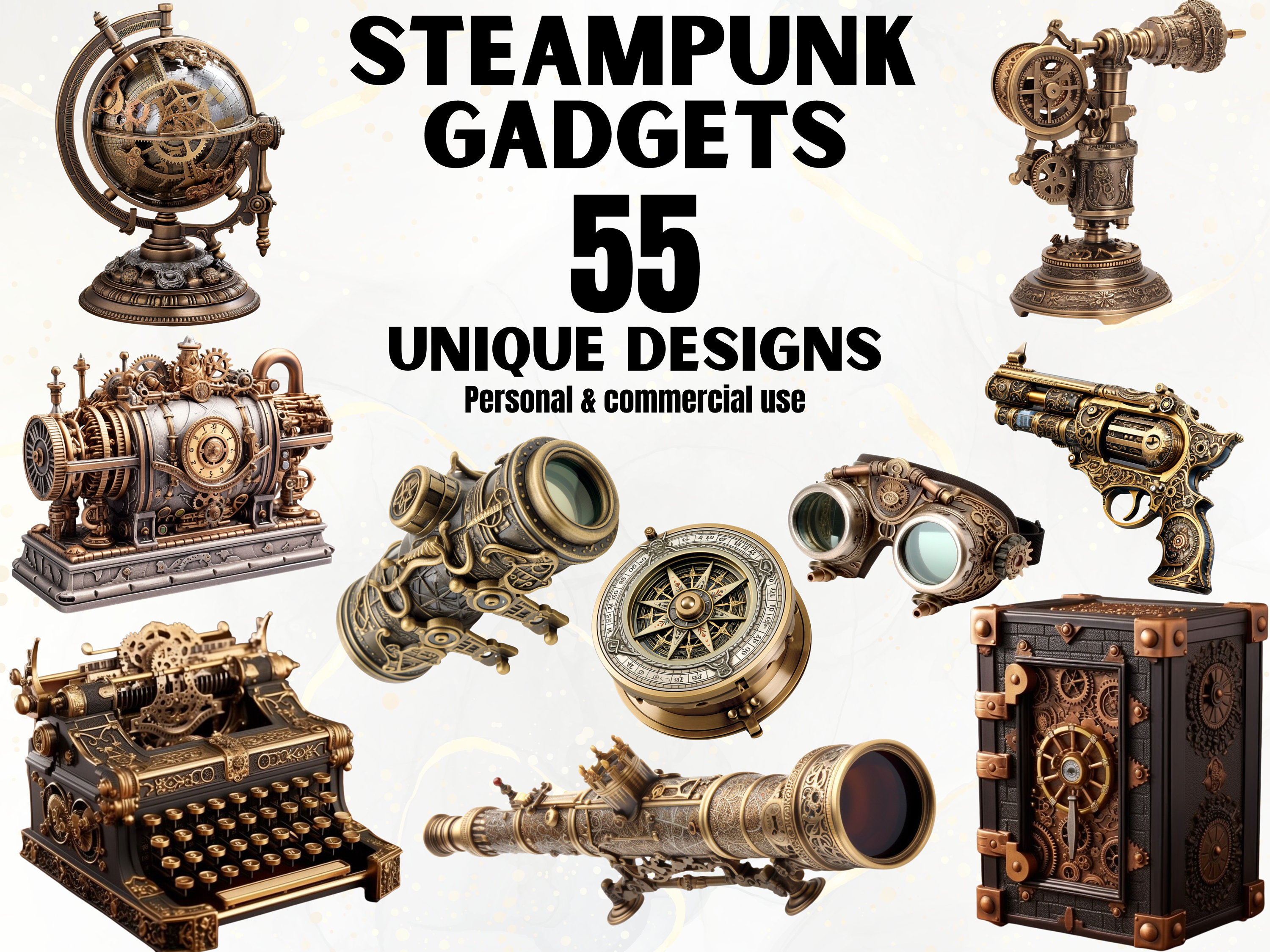An advertisement on a white background showcases "STEAMPUNK" prominently in capital letters at the top center. Directly beneath, it reads "Gadgets," followed by the number "55" and then "Unique Designs." The description continues with "personal and commercial use" in lowercase letters. The image is comprised of various steampunk-themed items. On the left side, from top to bottom, there's a globe, an ambiguous gadget featuring a clock, and a typewriter. On the right, from top to bottom, the items include a monoscope, a gun (specifically a revolver), and a safe. Adjacent to the safe, there's another monoscope, while in the top left corner of the safe, there are goggles without straps. The items are described as intricate designs made from brass, with gold accents and gears, embodying the steampunk aesthetic.